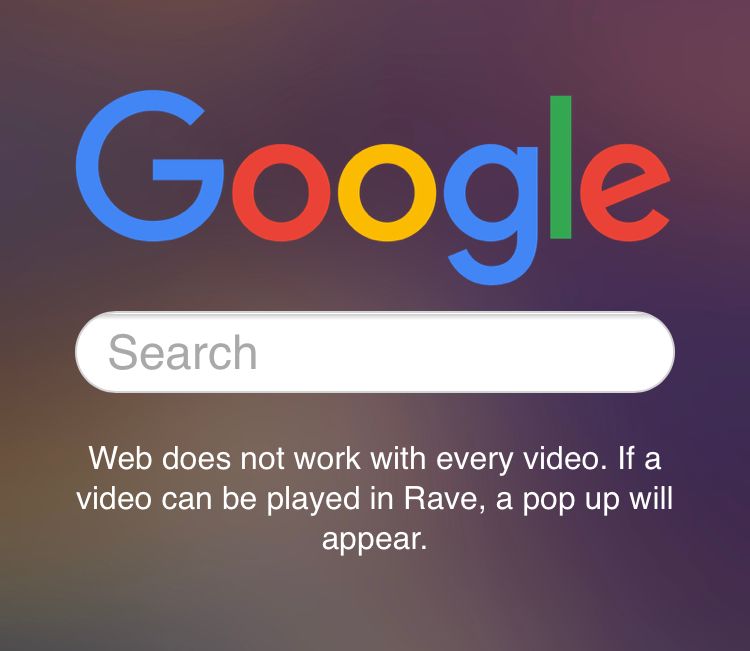This image closely mimics the familiar Google search page interface, potentially as a mock-up. At the top, the iconic Google logo is prominently displayed, with the letters "G", "O", "O", "G", "L", and "E" colored in blue, red, yellow, and green respectively. Below the logo, a classic search bar features placeholder text that reads "Search."

Underneath the search bar, there's a notice that reads: "Web does not work with every video. If a video can be played in Rave, a pop-up will appear." This notice adds a specific context related to the Rave app.

The design captures attention with its elements, particularly the logo and the search bar, while the background remains blurred to emphasize these main features. The layout and typography closely replicate the well-known Google search interface, with an added focus on the informative text related to video compatibility with Rave.